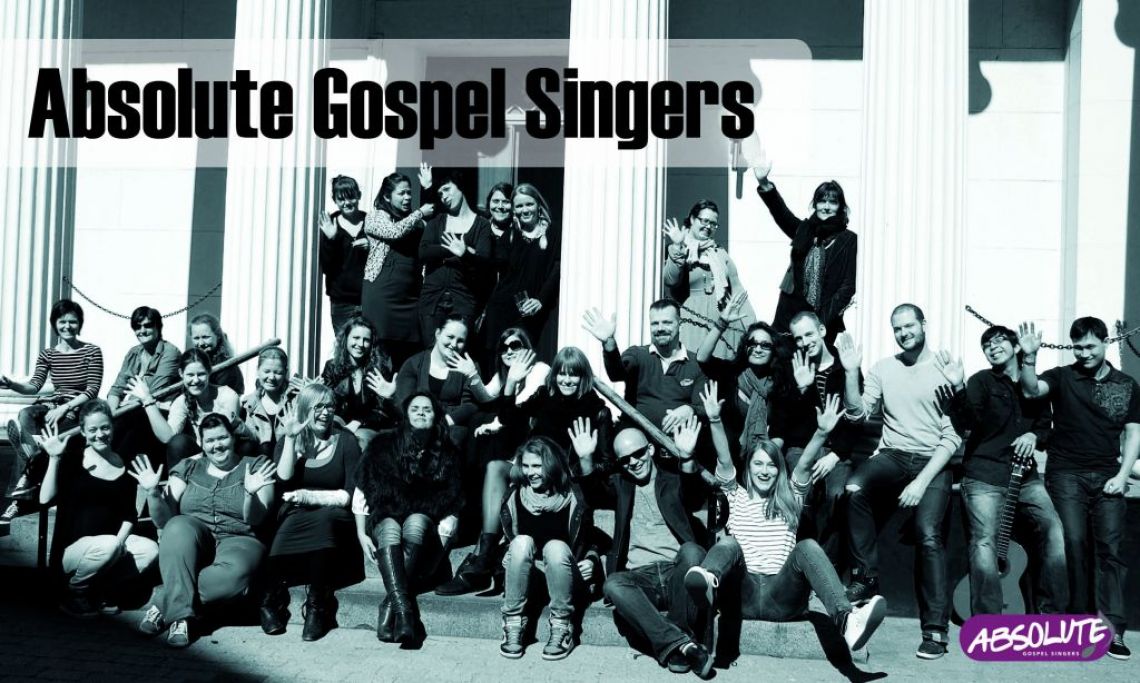The image is a black and white poster featuring a large group photograph of the Absolute Gospel Singers. This horizontal, rectangular image shows more than 50 men and women dressed in various casual clothes, arranged on the front steps of a building with prominent white column pillars, suggesting it was taken on a sunny day as shadows of the columns are visible. There are three rows of people: two seated rows and a standing group at the back. The people in the photo display a sense of unity and camaraderie. At the top left, the group's name, "Absolute Gospel Singers," is boldly printed in large black letters on a whitish background. Towards the lower right corner, a purple oval encloses the word "absolute," serving as the logo of the singing group. This visually striking photo captures the collective spirit and identity of the Absolute Gospel Singers.